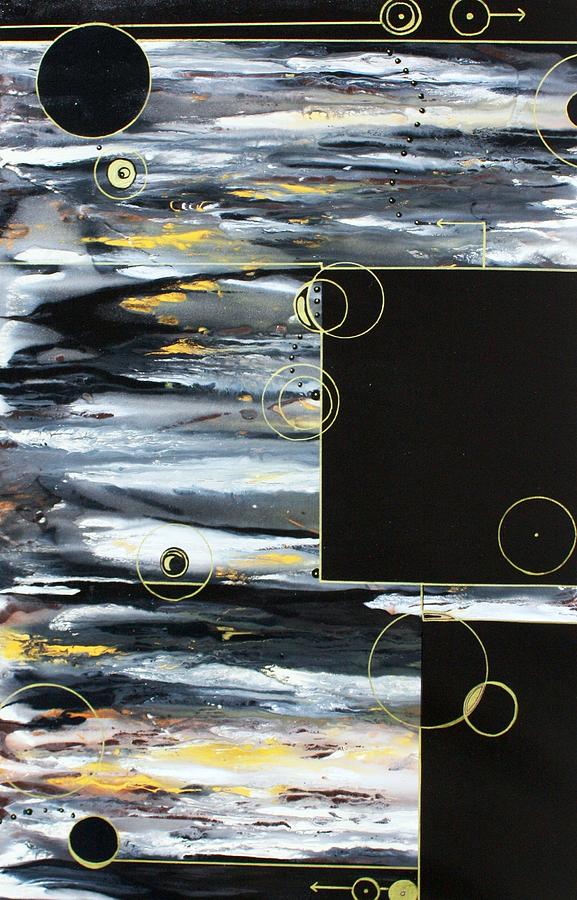This image depicts an abstract painting of a desolate, otherworldly surface. The composition features a background dominated by shades of grey, white, and a rusty yellow, giving the impression of an uninhabited planet. In the top-left corner, a prominent black circle, outlined in yellow and dotted with tiny white spots, stands out. The artwork is interspersed with several yellow circles of varying sizes, seemingly random and enclosing different parts of the painting for unclear reasons. The central right side of the image showcases a large black rectangle bordered by a yellow outline, while a smaller black rectangle is situated in the bottom-right corner. The painting also displays grayish, whitish, and yellowish streaks, resembling waves, with some sections containing a mix of orange streaks. The streaks and patterns repeat in different segments, contributing to the layered complexity of the artwork.